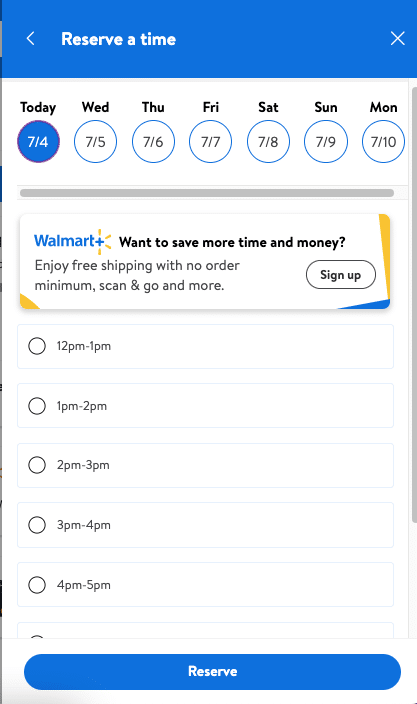Screenshot of a phone screen displaying a reservation page. The top part features a light blue bar with bold white text that reads "Reserve a Time", accompanied by navigational buttons to go back or exit. Below, a strip of dots separates the top bar from the main content. The main content area displays days of the week in bold black letters on a white background: Today, Wednesday, Thursday, Friday, Saturday, Sunday, and Monday, alongside corresponding dates: July 4th to July 10th.

The screen continues with a gray bar containing a promotional blurb for Walmart. The Walmart logo in blue, followed by a bold black text asks, "Want to save more time and money?" In lighter gray or light black text, it promotes benefits such as "enjoy free shipping with no order minimum, scan and go, and more." There is an option to sign up through a clickable button.

Below this blurb, a reservation interface displays available time slots: 12 to 1 p.m., 1 to 2 p.m., 2 to 3 p.m., 3 to 4 p.m., and 4 to 5 p.m. No time slot has been selected yet. Users can choose a time slot and click "Reserve" to confirm their selection.